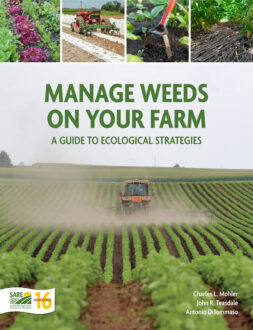The cover of the book titled "Manage Weeds on Your Farm: A Guide to Ecological Strategies" presents a montage of vibrant and instructive imagery related to farming. Nestled at the top of the cover are four smaller images: the first depicting an abundance of fruit, the second showing a tractor at work, the third illustrating a gardening hoe digging into the soil, and the fourth featuring what appears to be a bundle of shrubs or sticks. Below these images, the book's title is prominently displayed in green letters, occupying the upper third of the cover against a backdrop reminiscent of a clear sky.

The lower two-thirds of the cover feature a detailed and picturesque vista of a farm. Rows of green crops stretch towards the horizon, creating a serene and orderly landscape. A tractor, highlighted in different photos as both yellow and red, is seen actively plowing through the fields, churning up dust and debris, which adds a dynamic sense of movement to the scene. The dirt pathways between the rows of crops are distinct, and details such as a shovel and plastic sheeting used for weed control are also visible, highlighting the book’s practical approach to sustainable farming.

At the bottom left corner of the cover, there is a small logo that reads "SARE 16," signifying a possible affiliation or endorsement. To the right of the logo, the names of the three authors are listed in white letters, though they are somewhat difficult to make out: possibly Charles L. McFerrin, John R. Tersedale, and Antonio da Romano. The overall color palette of the cover image is dominated by earthy greens and browns, complemented by hints of pink, creating an inviting and informative visual guide to ecological farming strategies.